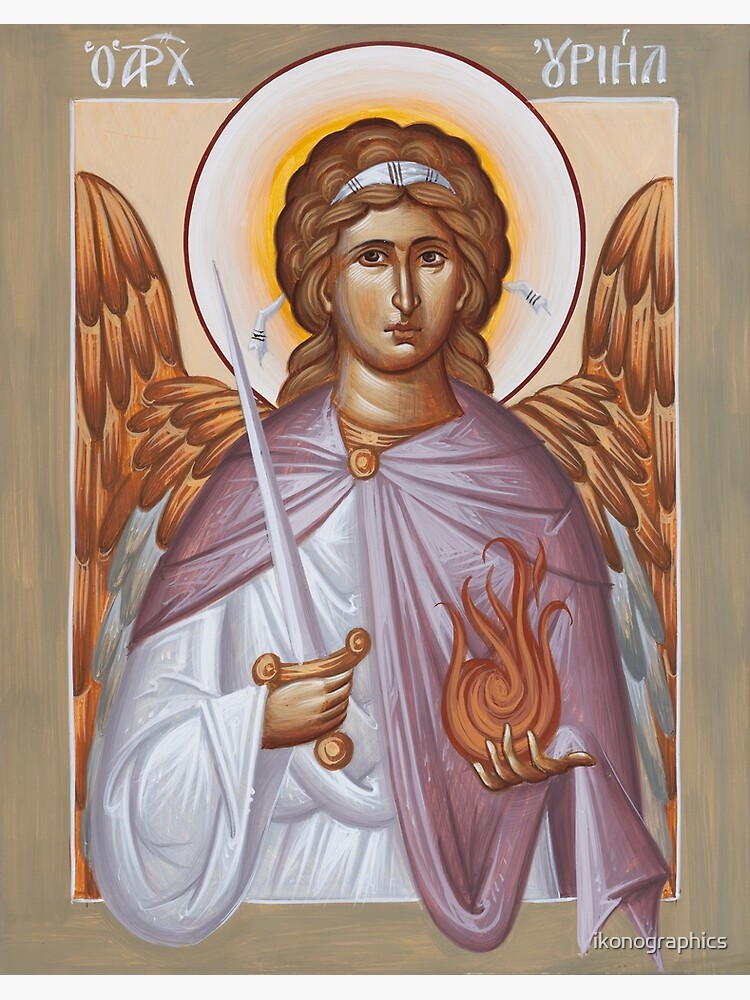This image depicts a spiritually themed illustration resembling a saintly figure or angel, characterized by an ethereal and majestic presence. The angel is adorned in a flowing white robe, which is complemented by a purplish cape draped over the left shoulder. This cape is fastened with a single button, adding to the regality of the figure. 

The angel's long, wavy brown hair is meticulously tied back with a strip of white cloth, further enhancing the serene appearance. A halo, initially gold at the base and transitioning into white and then brown, envelops the angel's head, surrounded by a faint yellow glow, illuminating a sense of divinity.

In the right hand, the angel grasps a gleaming sword, while the left hand holds a vibrant fireball, suggesting a dynamic and powerful nature. The wings, an intricate blend of white and gold feathers, spread gracefully from the figure's back, emphasizing the celestial theme of the scene.

Text adorns the top of the card, written in an enigmatic script that could be Greek or a stylized, fictional creation to match the tarot card-like aesthetic. Additionally, the bottom right-hand corner features the text "Icon Graphics," spelled as "I-K-O-N-O-G-R-A-P-H-I-C-S," indicating the graphic design origin of the illustration.

The entire image is framed by a brown border, resembling a picture frame, adding a classic and finished look to the artwork, which one might expect to find displayed within a church setting.